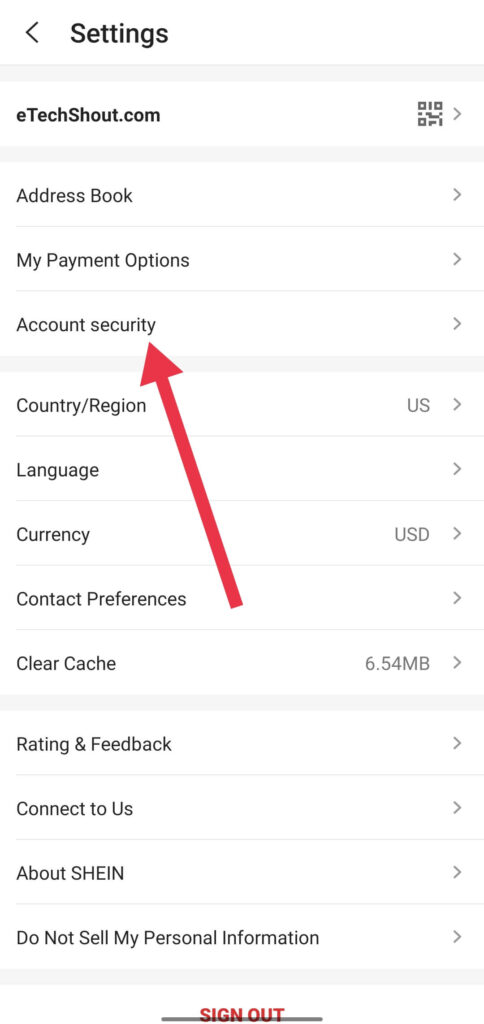This image appears to be a screenshot taken from a cell phone displaying the settings menu of a website identified as etechshout.com. The menu items are listed along the left side of the screen. At the top, the website's name "etechshout.com" is prominently displayed. Directly below, the following options are listed in sequence: "Address Book," "My Payment Options," "Account Security," with a noticeable red arrow angled upward pointing to "Account Security."

Further down, a thin gray line separates "Account Security" from the subsequent categories: "Country/Region," "Language," "Currency," and "Contact Preferences." Following these are "Clear Cache," another separated by a thin gray line. The next set of items includes "Rating and Feedback," "Connect to Us," "About Shein," and "Do Not Sell My Personal Information." At the bottom of the menu, in bold red capital letters, the option to "SIGN OUT" is clearly displayed, indicating the logout function.

This description captures all visible segments and elements within the displayed settings, emphasizing key details for clarity and completeness.